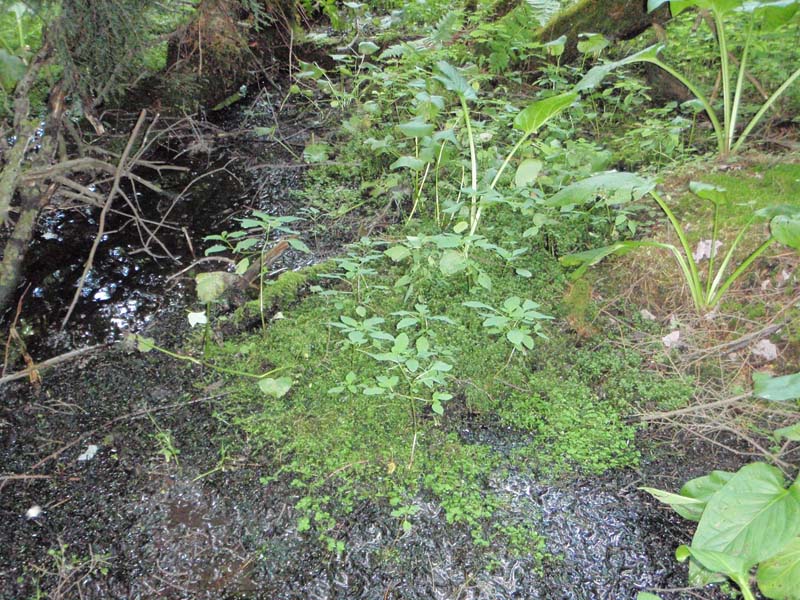This outdoor daytime image captures a serene forest scene with lush foliage and abundant greenery. A tranquil creek, visible on the left side of the image, flows from the middle left towards the top, with light glistening on its surface, indicating sunlight. The creek is bordered by a moss-covered, gray bank dotted with various plant life. Exposed tree roots are visible on the bottom left, emerging from the ground, creating a dynamic texture alongside rocks scattered on the dirt ground. The right side of the image showcases a variety of green plants and leaves, including broadleaf plants and low-growing greeneries, which further enhance the verdant atmosphere. Fine branches, possibly from nearby bushes, slightly overhang the creek, adding an intricate detail to the natural setting.